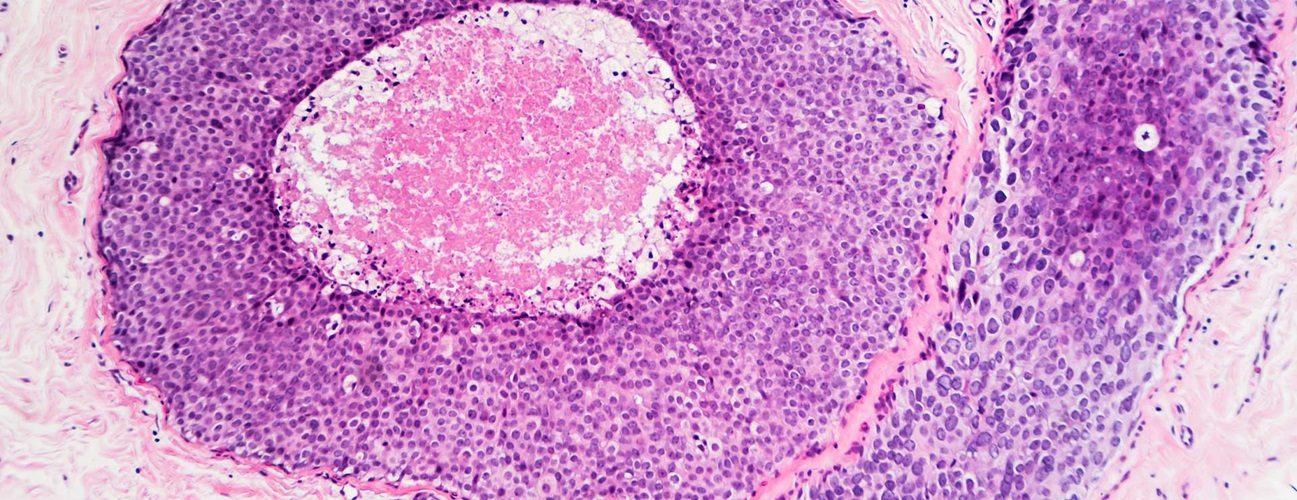This rectangular image, possibly a painting or a microscopic close-up, features an organic, textured appearance with a multitude of colors and patterns. Dominating the image is a large, donut-shaped formation on the left, filled with dense clusters of purple and pink specks resembling fine cellular patterns. The center of this donut-like shape has white and pink spots that evoke the texture of marble or granite. The background is predominantly white, providing contrast to the vivid colors. On the far right, a similar cluster of purple specks forms an angled line, also surrounded by a white and pink fluid-like backdrop. The overall effect is one of intricate, organic detail, whether it be an artistic creation or an enlarged microscopic view.